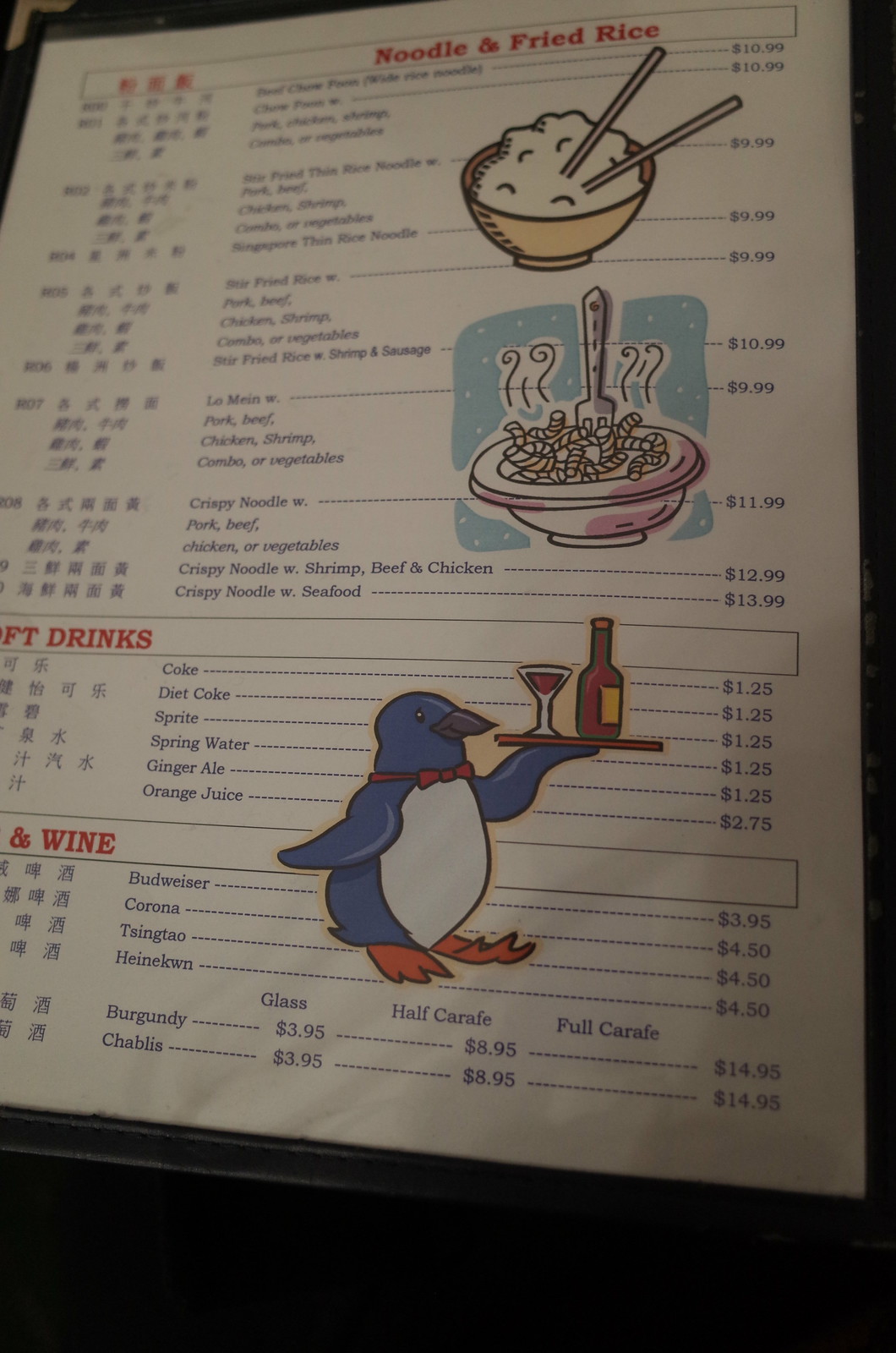This image depicts a restaurant menu prominently featuring noodle and fried rice dishes at the top. The menu is largely written in Chinese characters, which are unreadable to non-Chinese speakers. Smaller English text is also present but not clearly visible. Listed prices for the dishes start at $10.99, followed by various items priced at $9.99, $11.99, $13.99, and $1.25. The menu also highlights sections in red text for "Soft Drinks" and "Wine." An illustration of a penguin, dressed as a waiter, carries a tray with a cocktail and a beer bottle, adding a whimsical touch to the otherwise minimalistic design. The background of the menu is plain white.